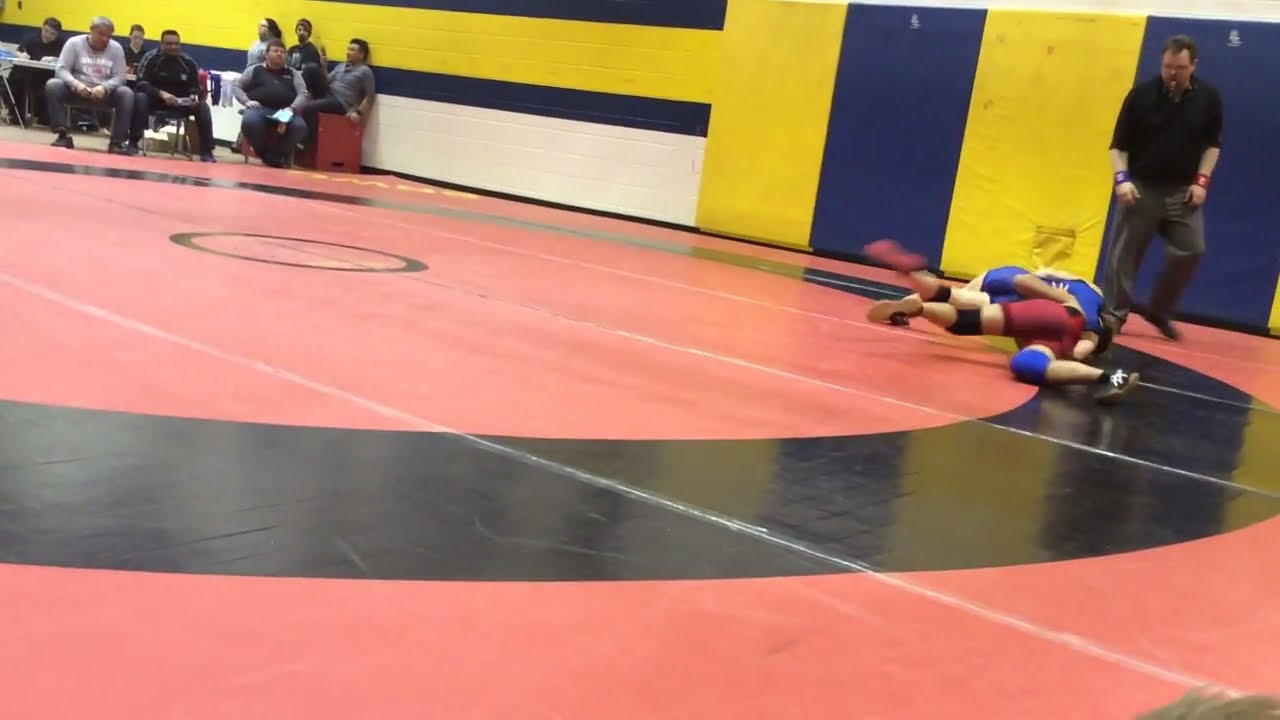This image portrays a high school wrestling match taking place inside a gymnasium. Centered on a red wrestling mat, with a crowd of spectators visible in the background, two boys face off, each dressed in knee guards and black sneakers; one wears a red uniform and the other a blue one. Behind them, a large banner is prominently displayed on the wall, reading "Pride and Tradition" in both English and a second language, presumably Spanish or French. Signage at a judge's desk in the foreground mentions "Ontario Mat Tapas 1," indicating either location or sponsorship. The gym's decor includes blue and yellow line patterns, and a camera on a tripod is set up near the desk, capturing the event.